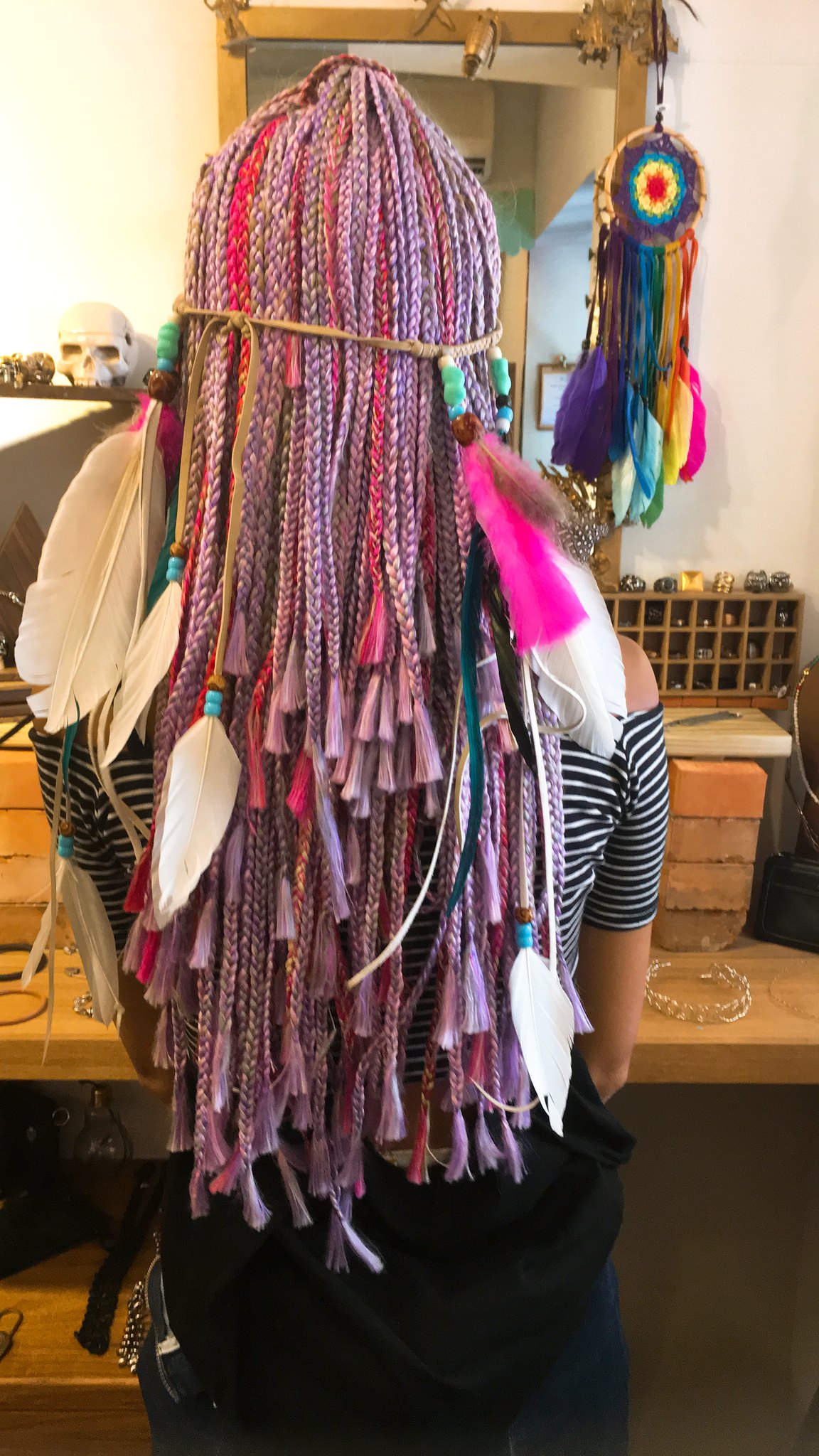The photograph captures a detailed and vibrant scene set indoors, focusing on a woman viewed from behind. She stands in front of a large mirror with a brown frame, adorned with a colorful dreamcatcher. The dreamcatcher's circular centerpiece features a red sun surrounded by bands of yellow, green, and purple, with an accompanying tail in similar shades of purple, green, blue, orange, and pink.

The primary subject, a lady of small stature, wears a distinctive and intricate braided headdress. Her long hair, cascading down to her lower back in various lengths, features primarily lavender braids interspersed with bright pink ones. Some of these braids end in tassels, while others have white feathers attached. She also wears a thin, light tan strip of fabric or leather around her head, embellished with beads and additional feathers, including a notable hot pink one on the right side.

Her outfit consists of a black and white horizontally striped top, paired with blue jeans. The setting includes a wooden desk behind her, strewn with various pieces of jewelry and small items, and a shelf to her left that holds a skull. The meticulous detailing in both her hairstyle and the surrounding elements creates a richly textured and visually engaging image.